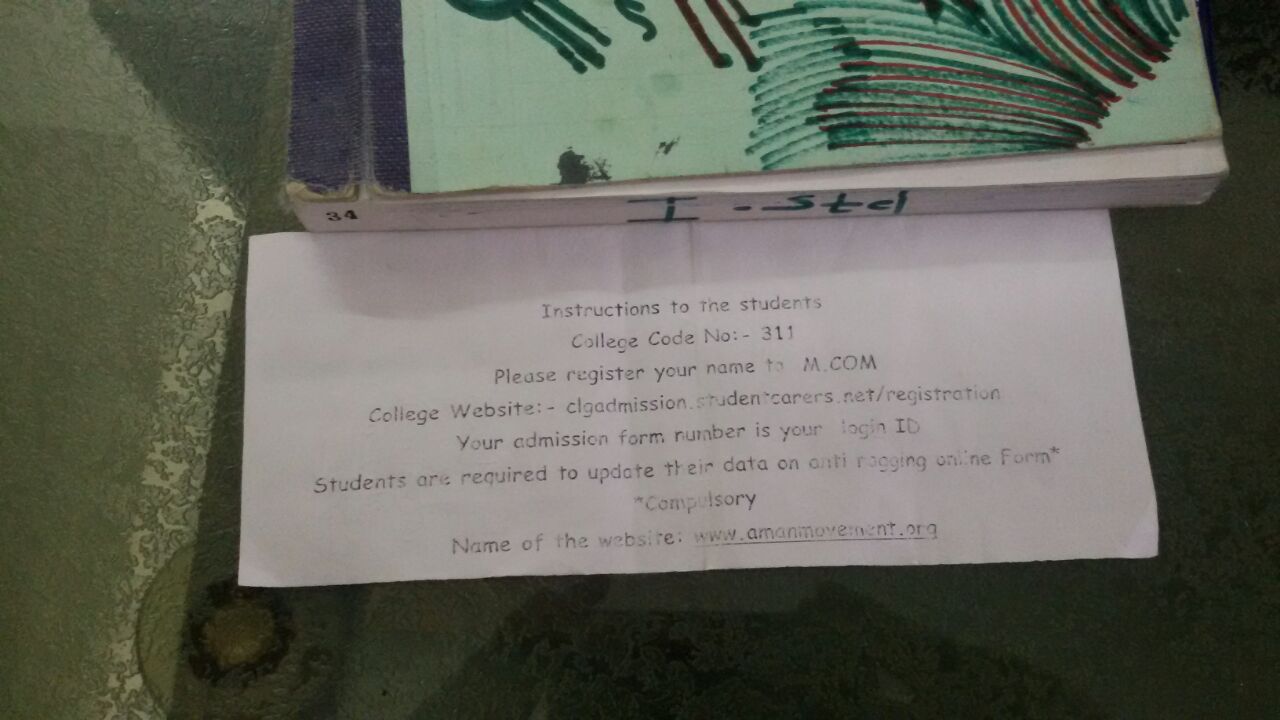The image features a rectangular box with a green design on its top, positioned prominently on a dark black table. Below the box, a white sheet of paper is spread out, occupying most of the visual focus. This paper contains detailed instructions directed at students, including the college code, registration guidelines, website information, the admissions contact number, and specific student requirements. Additionally, the document concludes by providing the name and URL of the relevant website. To the left of the table, a linoleum floor with a green pattern is partially visible.